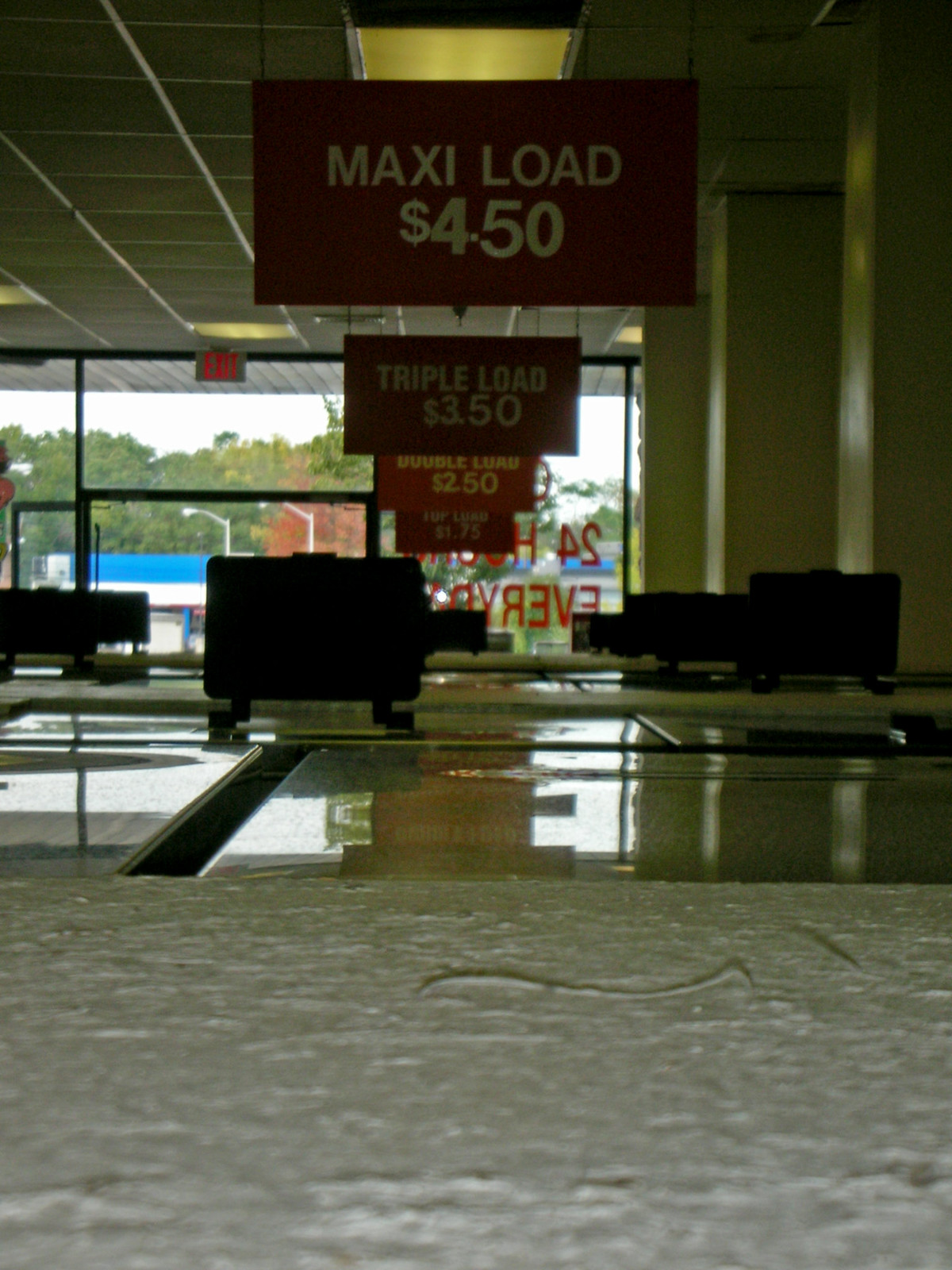The image depicts the interior of a building, with a detailed foreground and background. In the bottom section of the image, a gray structure is visible, likely a countertop given its elevated position above the floor. The floor beyond this countertop appears reflective, capturing white light and creating mirrored surfaces. Centrally positioned is a brown structure that also reflects on the floor, which is consistent across the left side as well.

In the background, tall black cases resembling briefcases are visible, with one prominently positioned in the left center and another on the far right. There are several red signs with white text, indicating various load capacities: "MAXI LOAD 450," "TRIPLE LOAD 350," and "DOUBLE LOAD 250."

Further behind, a row of windows allows natural light to filter in, revealing an exterior scene of a light blue building and a collection of trees, providing a serene backdrop to the bustling interior.